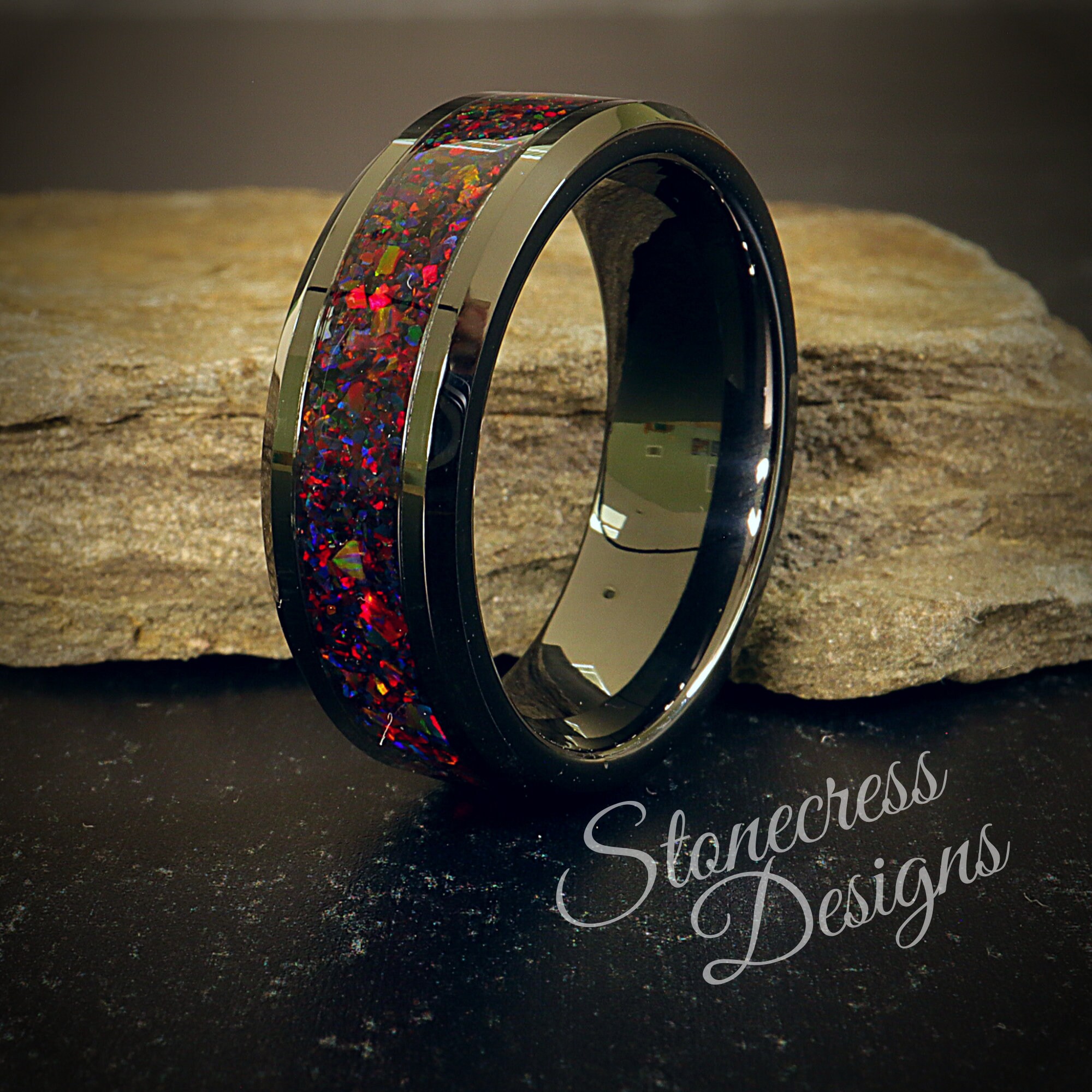The image features a colorful and creatively designed metallic ring, which appears to have a confetti-like interior filled with tiny specks of vibrant colors, including bright red, pink, blues, purples, green, yellow, and a blackish-gray. The ring, positioned directly in the middle and slightly tilted towards the left, is prominently displayed to showcase its unique design and intricate details. Just behind the ring is a stone, adding to the overall aesthetic of the image. In the bottom right corner, white and gray text reads "Stoneness Designs," indicating the maker of the ring. The background features a light, stonish grayish beige color, complementing the ring's vivid colors and enhancing its visual appeal. The positioning and detailed display of the ring, along with the text, suggest a focus on high-quality design and craftsmanship from Stoneness Designs.